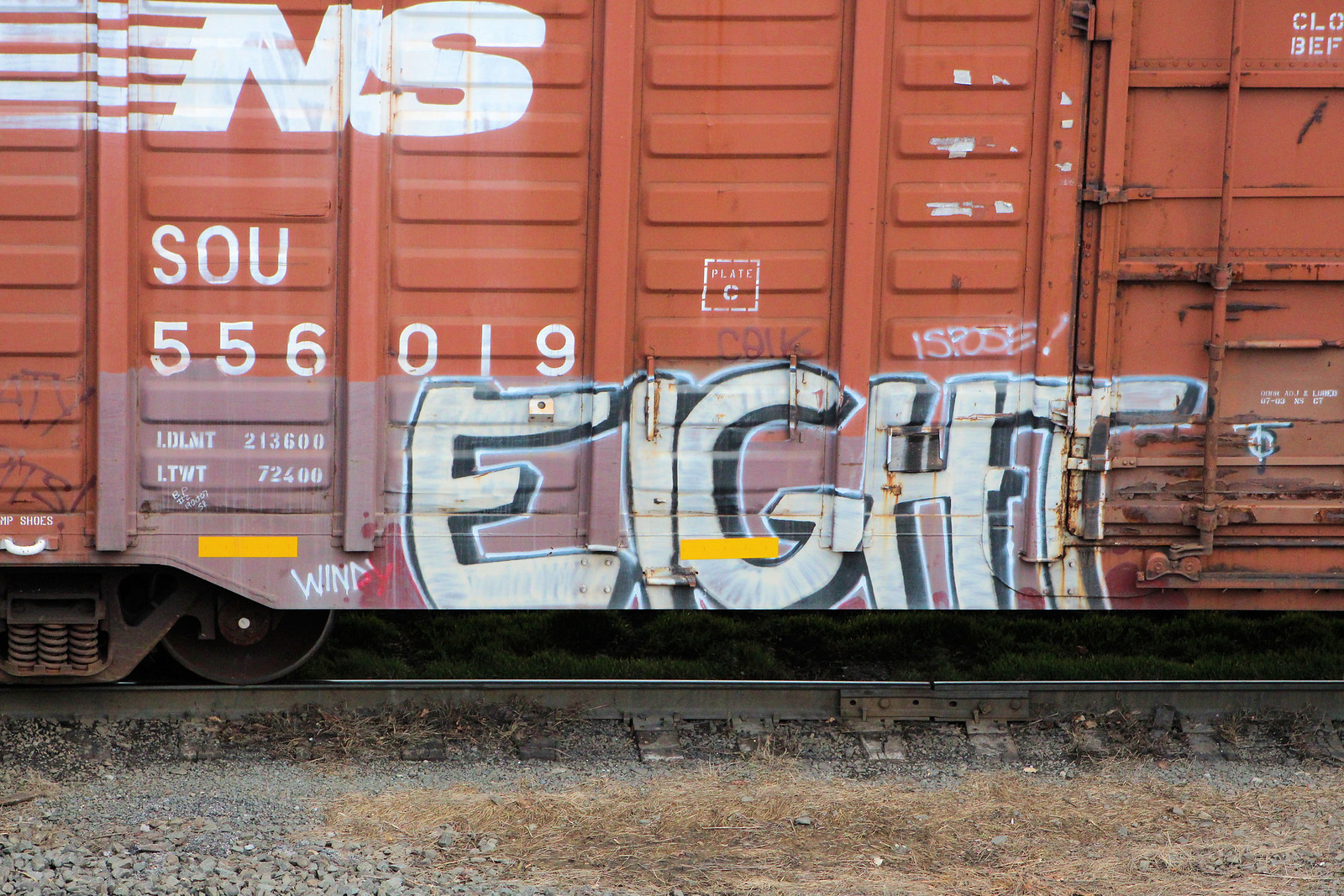This image captures a detailed close-up of a Norfolk Southern boxcar with the number SOU556019. The boxcar, a rusty burnt orange, rests on railroad tracks surrounded by gravel and patches of dead grass. Prominently displayed in the top left corner is the Norfolk Southern logo, featuring the capital letters "NS" adorned with five white stripes on the left side of the "N". The car also bears a square label in the center, with the letters "P-L-A-T-C" and a smaller 'C' above it. Both the wheels and gears are notably rusted. Adding a striking element to the scene is the graffiti on the lower part of the boxcar, where the word "8" is painted in white bubble letters. These letters are highlighted with a black band, which in turn is outlined with a thin white band, giving the graffiti a three-dimensional appearance.